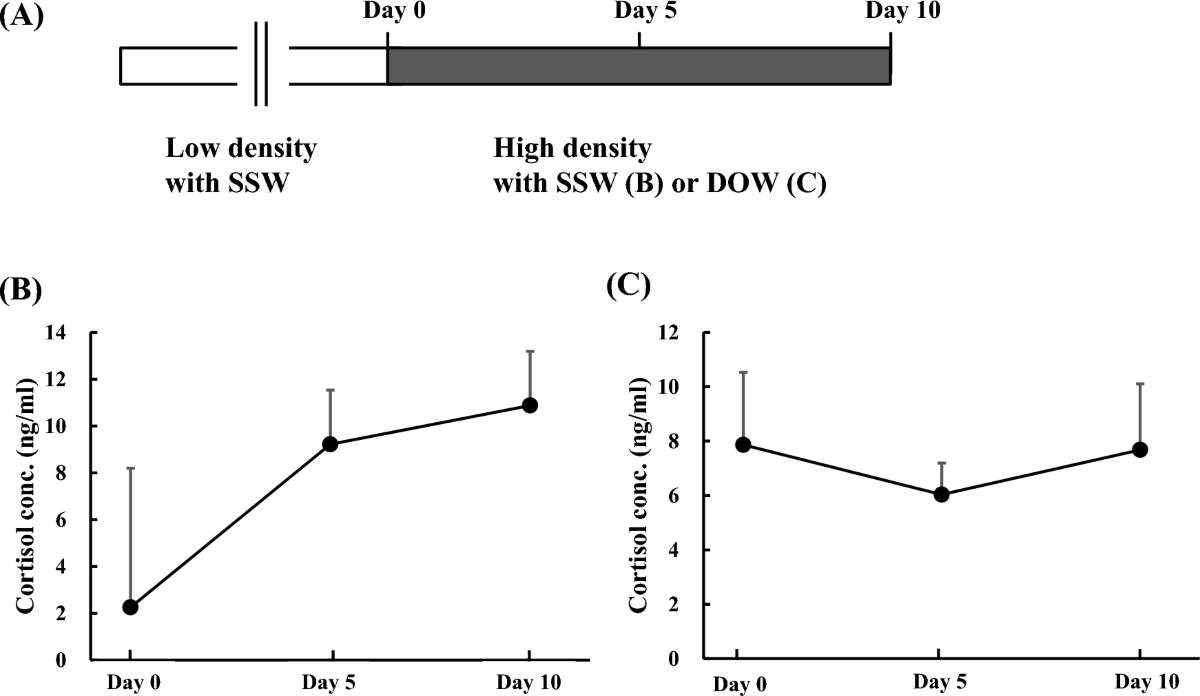The image features a set of three diagrams, each with distinct graphical elements printed in black on a white background. 

At the top lies a horizontal bar divided into two sections: a white section labeled "Low Density with SSW" and a black section marked "High Density with SSW or DOW," stretching from day 0 through day 10. 

Below this are two separate X-Y graphs. Both graphs have the days indicated on the X-axis, spanning from day 0 to day 10. The Y-axis of each graph measures cortisol concentration (C-ON-C or CUNC). The left graph illustrates an ascending trend in cortisol levels, starting around 2 and rising to approximately 10 by day 10. In contrast, the right graph shows more variability with cortisol levels starting at around 8, dipping to 6, and then returning to 8, indicating a fluctuating pattern.

Overall, the image clearly delineates variations in cortisol concentration under different density conditions across a timeline of 10 days.